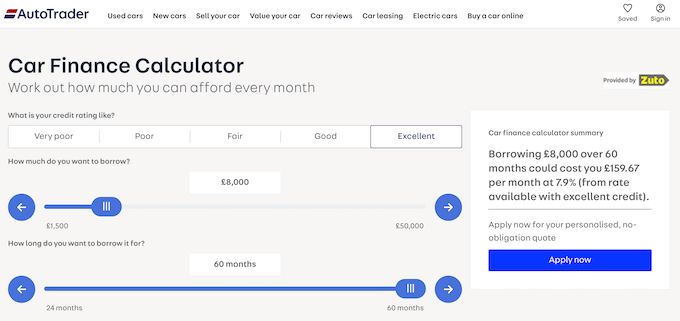This is a detailed screenshot of the Autotrader website, captured from a desktop or laptop computer. In the upper left corner, the distinctive Autotrader logo is prominently displayed. The logo features a flag motif with three horizontal stripes: red at the top, white in the middle, and blue at the bottom. Adjacent to the logo, "Autotrader" is written in black font.

To the right of the logo, there is a series of horizontal header tabs. These are, from left to right: "Used Cars," "New Cars," "Sell Your Car," "Value Your Car," "Car Reviews," "Car Leasing," "Electric Cars," and "Buy a Car Online." Each tab serves as a navigation option for different sections of the website.

In the upper right corner of the page, two icons are featured: a heart symbol, which represents saved items, and an icon resembling a human head enclosed within a circle, indicating the sign-in button.

The main body of the website is rectangular with a gray background. The heading "Car Finance Calculator" is written in black lettering. Below it, the subtitle reads, "Work out how much you can afford every month." The page includes input fields for users to enter details such as their credit rating and the amount they wish to borrow. The currency used on this website is British pounds, indicating that the website caters to users in the UK or those dealing with UK currency. The remaining text is in blue font, providing a clear and legible interface.